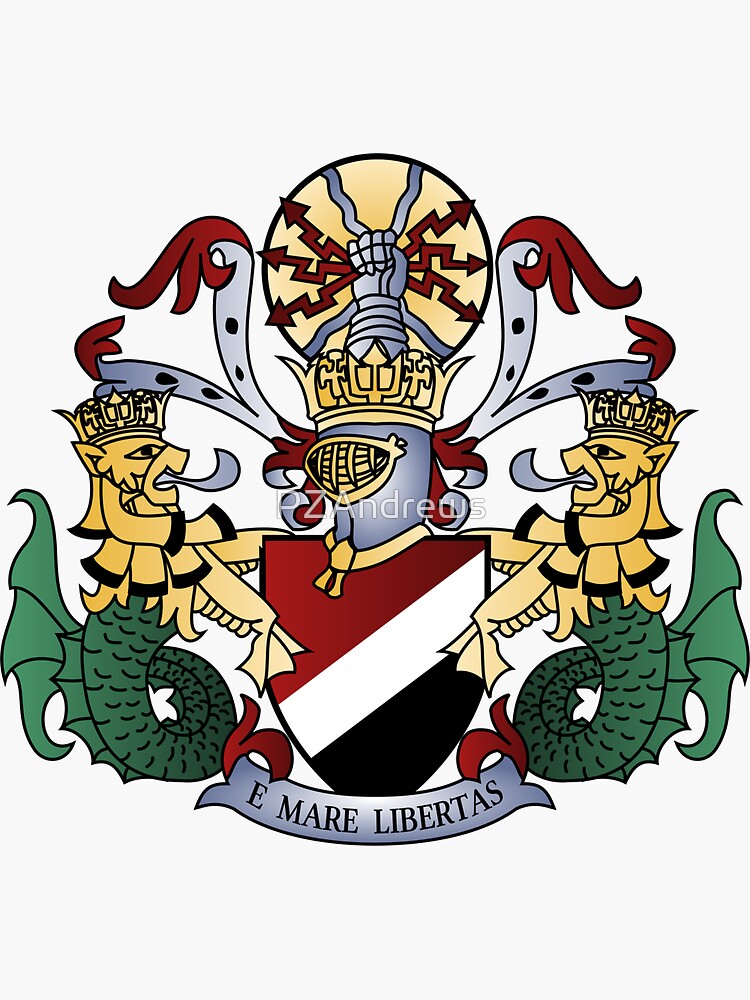This detailed, color illustration in portrait orientation depicts a coat of arms with intricate heraldry. Central to the composition is a shield adorned with diagonal stripes in red, white, and black. Flanking the shield are two crowned lions, each featuring a mermaid-like tail, colored in green. Both lions face each other, symbolizing guardianship and symmetry. Above the shield, a knight's helmet also sporting a crown supports a clenched fist holding six red arrows, adding a martial element to the design. At the very top, a yellow circle with a black outline and gold filling adds further distinction. Flourishes in gray and red embellish the sides, enhancing the overall ornate appearance. Below the shield, a scroll banner bears the Latin text "I Mare Libertas" in black ink. The background is a light gray, allowing the vivid colors and detailed line art to stand out prominently.